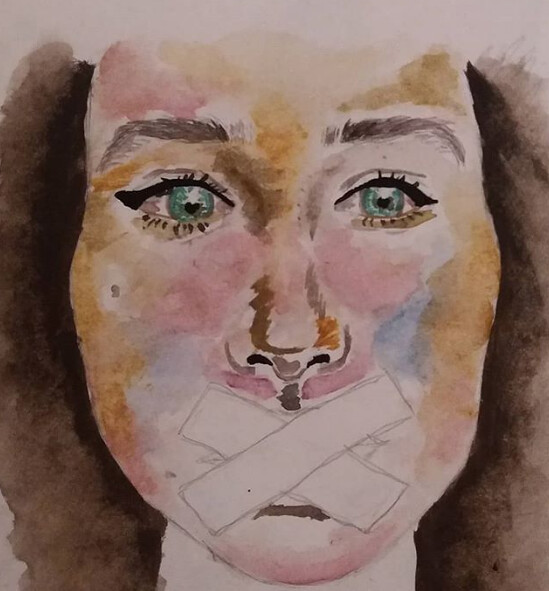The image, resembling a painting created with markers, depicts a close-up of a woman's face. She has striking green eyes with thick eyebrows, which appear dark and defined, accentuated by black eyeliner. The woman's face is painted in various shades of brown and pink, with hints of blue and purple around her nose and cheeks. Her brown hair frames her face on the left and right, though the top of her head isn't visible as it's left unpainted, showing white. Distinctively, her mouth is covered by two strips of tape arranged in an X shape, lending the image a speechless quality. The background is a pinkish hue, further emphasizing the detailing in the woman's expressive and muted visage.